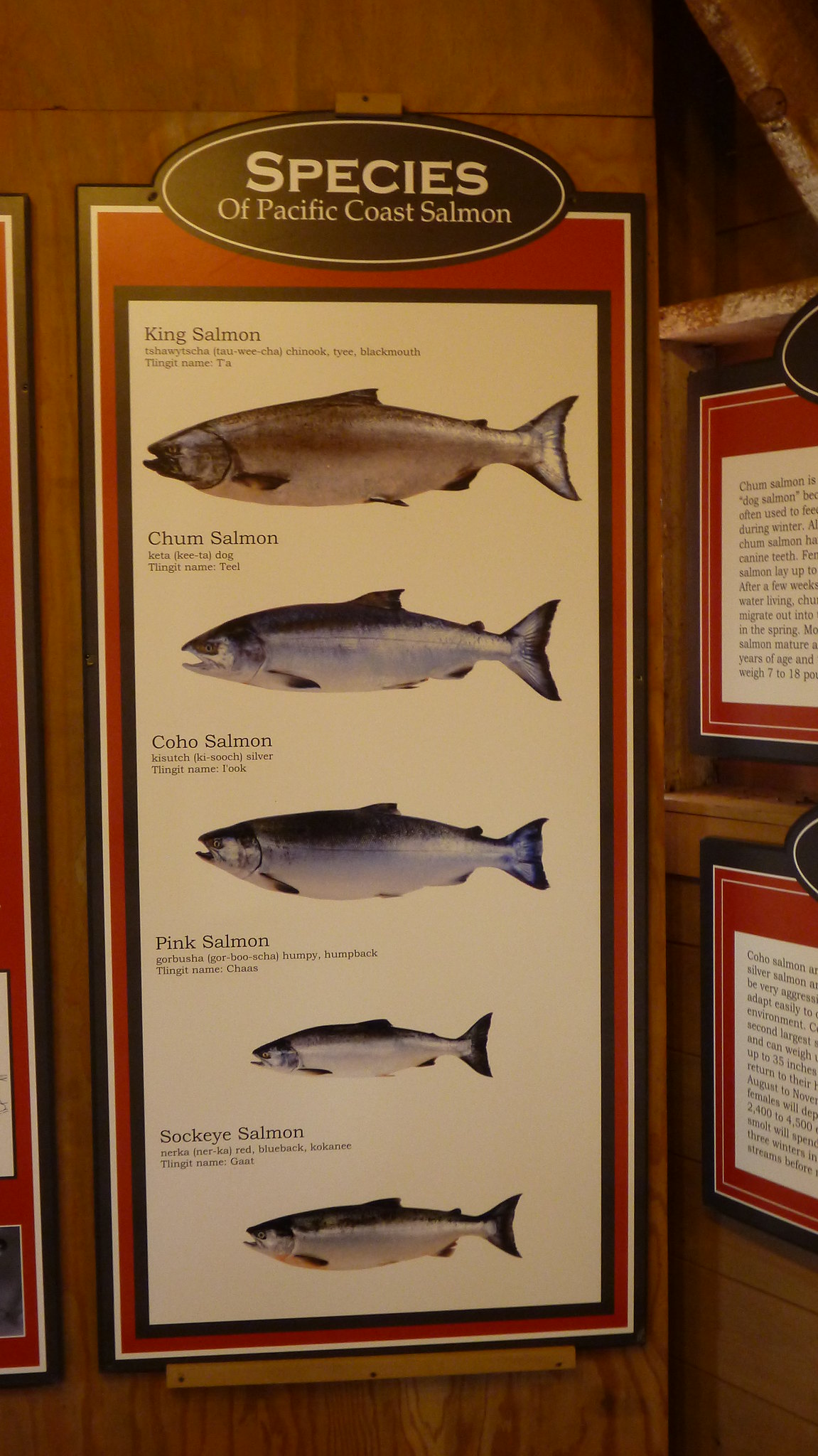This image showcases a detailed, framed collection of illustrations and descriptions of various Pacific Coast Salmon species, prominently titled "Species of Pacific Coast Salmon" in white text on a black oval background. The framed display features multiple rows of detailed fish depictions, each accompanied by brief but intricate descriptions. At the top, the King Salmon (also known as Taweecha, Chinook, Tai'i, Black Mouth, and by its Tlingit name Ta) is illustrated, showcasing a brown and gray fish. Below it, the Chum Salmon (Kita Dog, Tlingit name Teal), with its grayish-blue hues, is depicted. Next, the Coho Salmon (Kisook Silver, Tlingit name Took) is illustrated in silver and blue shades, slightly rounder at the bottom. Continuing down, the Pink Salmon (Gorbusha Humpy, Humpback, Tlingit name Chaas) is slimmer and similarly colored. At the bottom, the Sockeye Salmon (Nurka Red, Blueback, Kokani, Tlingit name Gat) features an orangish spot, transitioning to white and dark brown hues. Each fish's name and Tlingit name offer cultural insights into their significance. To the side, other framed writings and pictures, possibly containing narratives or additional details, are partially visible, hinting at a broader context for the collection. The entire display is mounted on a wooden paneled wall, adding a rustic touch to the informative exhibit.